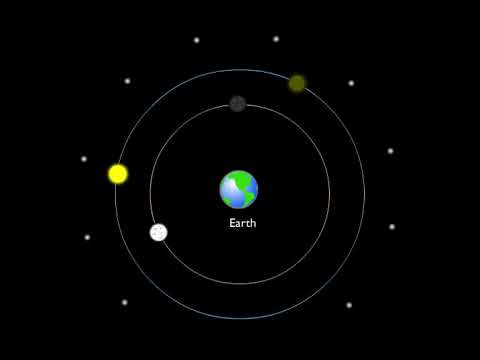A rudimentary diagram of our solar system is set against a plain black background. At the very center of the image is a small, cartoonish depiction of Earth with vibrant blue water and green land masses, labeled "Earth" in white letters directly below it. Two rings encircle the Earth, indicating the orbits of various celestial bodies. 

On the inner orbit, there is a small black circle positioned directly above Earth and a pinkish-white circle next to it on the left. Additionally, there is a white dot, potentially representing the Moon. The outer orbit features a yellow circle to the right, likely the Sun, and a green circle above the black circle. Surrounding these orbits are numerous small white specks resembling stars. The diagram seems to illustrate how different celestial bodies might rotate around Earth or how they are positioned relative to day and night. There are other smaller dots scattered around, possibly representing additional planets or cosmic objects.